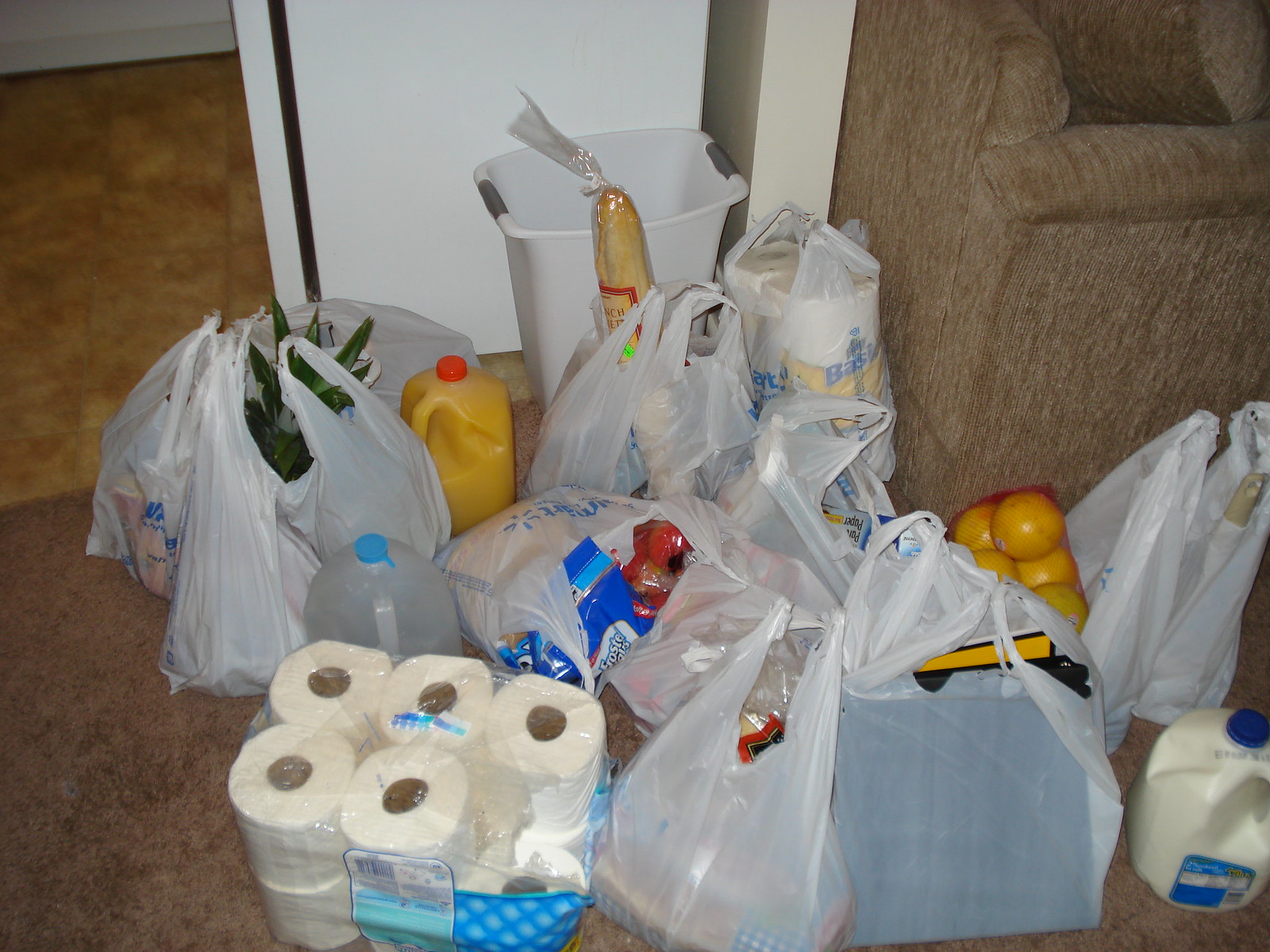The photograph, taken indoors, depicts a scene of groceries recently brought inside and placed on the floor. The floor has two distinct sections: a linoleum area in the background and a brown carpeted area in the foreground. On the carpet, there is a white wastebasket located near a couch. The groceries are mostly in white plastic bags, with a few items visible, including a gallon of milk with a blue label and cap, a gallon of orange juice, and a gallon of what could be water or vinegar. Other visible items are a loaf of French bread, a package of toilet paper, a two-pack of paper towels, a bag of chips, some citrus fruits like oranges or grapefruit, part of a pineapple, and some produce. The groceries appear to have been unloaded and set down next to what looks like the side of a refrigerator, with a wall partially visible behind it.